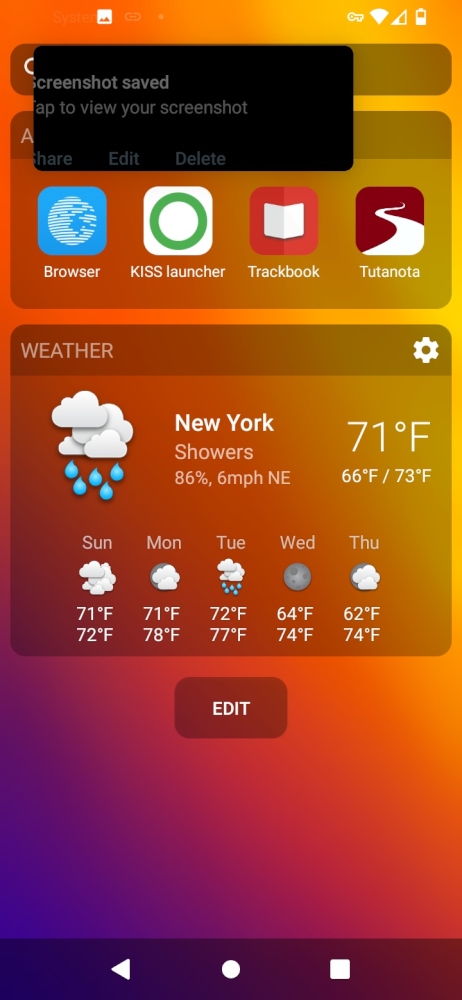The screenshot showcases a smartphone home screen enveloped in a gradient background transitioning from warm hues of orange at the top to a rich purple at the bottom. At the top of the screen, there's a notification banner stating that a screenshot has been saved, offering options to save, edit, and delete.

Beneath the notification banner, there is a grid layout featuring four application icons: a browser, the KISS launcher, Trackbook, and an app identified as Totonota, discernible by its icon featuring a white curve on a red background.

The prominent weather widget is located below these application icons, providing a detailed forecast for New York. Current conditions indicate storms or showers with a temperature of 71°F. Specific details include 86% humidity and a northeasterly wind blowing at 6 mph. Iconography shows a cloud with raindrops, symbolizing infiltrating showers. 

The forecast for New York is as follows: Showers on Sunday with a high of 72°F, Monday exhibiting 71°F low and 78°F high, Tuesday at 72°F low and 77°F high, Wednesday at 64°F low and 74°F high, and Thursday at 62°F low and 74°F high. An edit button is located at the bottom of the weather widget, allowing for further customization.